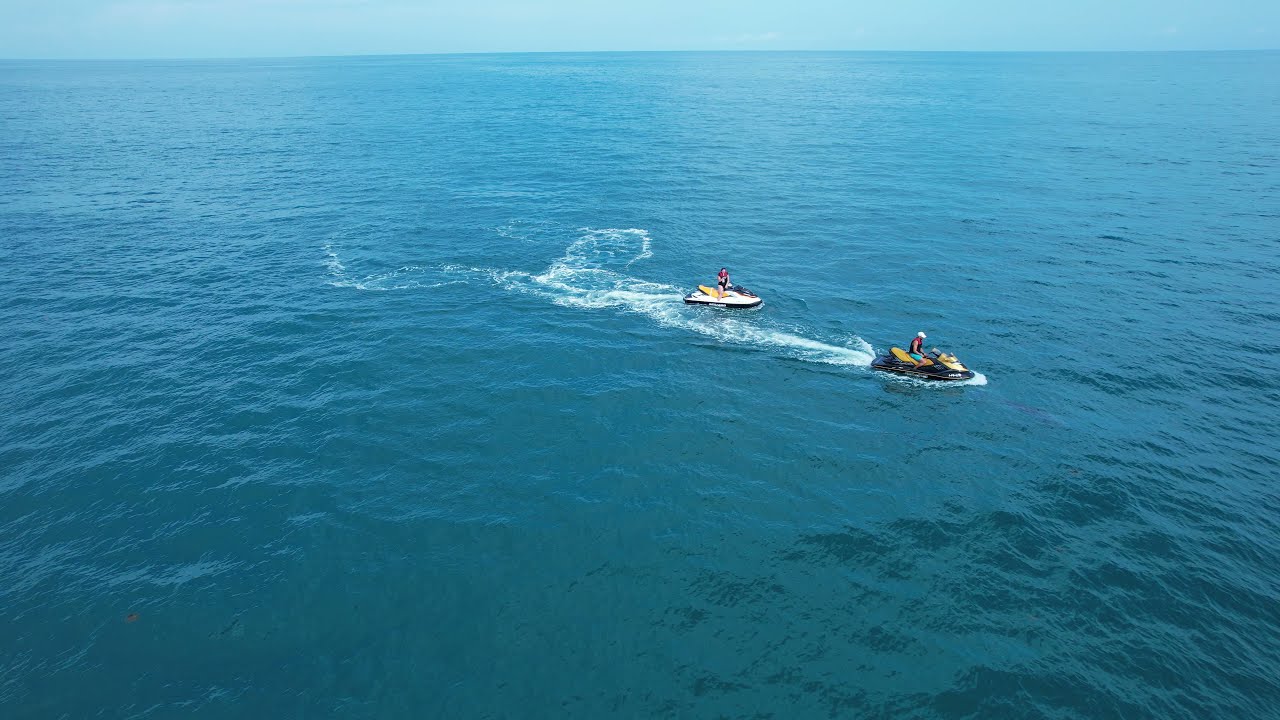This aerial daytime photograph captures a serene scene over the ocean, where two jet skis cut through the mostly calm waters, leaving gentle wakes behind them. The clear blue horizon stretches across the upper part of the image, transitioning from lighter to deeper shades of blue, emphasizing the vastness of the sea without any visible land. The two jet skis, one yellow and black and the other white and black, are positioned centrally in the frame, traveling from left to right. Each jet ski is piloted by a single rider wearing a life vest, with the lead rider in a dark blue shirt, light blue shorts, and a ball cap, and the trailing rider in a single-piece swimsuit, suggesting a female. The active motion of the jet skis is highlighted by the water trails they leave, adding dynamic energy to the tranquil ocean expanse.